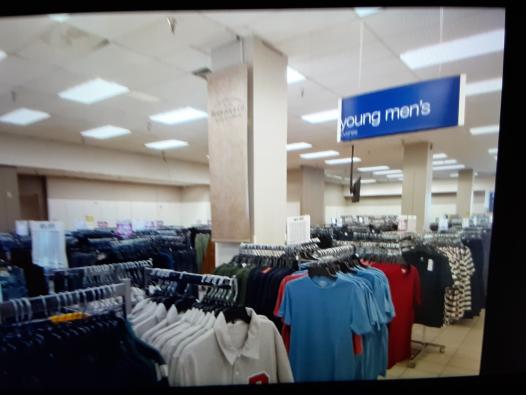The photograph captures the interior of a bustling department store, illuminated by rectangular fluorescent lights on the ceiling. A prominently displayed blue sign with white lettering reading "Young Men's" hangs from the ceiling, clearly marking the section. Centrally located within the store is a large support pole extending from the floor to the ceiling, adorned with a tan sign featuring a distinctive logo.

In the foreground, a clothing rack brimming with white collared shirts embellished with a red and white letter takes center stage. Directly behind this, another rack showcases a selection of vibrant blue t-shirts, with a row of red t-shirts further back. In the background, additional racks offer a variety of fashionable dresses, including striking red dresses, sleek black dresses, and eye-catching black and white striped dresses. The orderly arrangement of merchandise and the strategic signage create a welcoming and organized shopping environment.